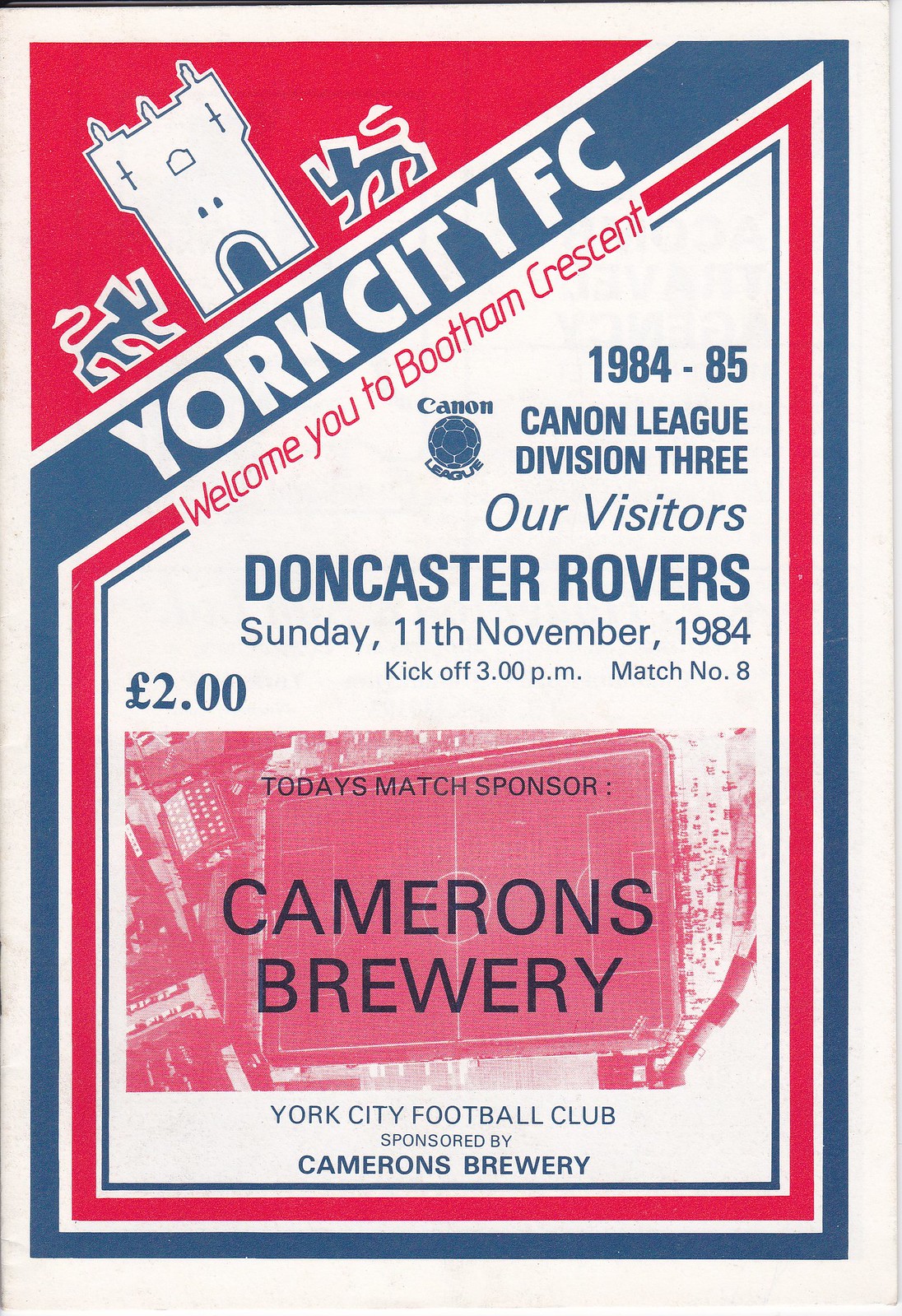This image is the front cover of a York City Football Club program for their match on Sunday, 11th November 1984. The background is cream with a prominent red triangle in the top left corner. Inside the triangle are two blue mythical creatures, possibly griffins or lions, flanking a white tower. Below the triangle is a blue border running parallel to its bottom edge and extending down both sides and across the bottom of the cover. Within this blue border, in white letters, it reads "York City FC."

Below the blue border, a red border states, "Welcome you to Bootham Crescent." Further down in blue text, the season "1984-85" is mentioned, along with a Canon League Division III logo featuring a soccer ball. It announces “Our visitors, Doncaster Rovers,” followed by the match details: "Sunday, 11th November 1984, Kickoff 3 pm, Match number 8."

A red-filtered photo of the football pitch is displayed with blue text overlaying it, "Today's match sponsor, Cameron's Brewery." At the very bottom on the white background, it reaffirms, "York City Football Club sponsored by Cameron's Brewery." This program is reminiscent of a ticket, detailed with advertisements, names, dates, and times, and is priced at £2.